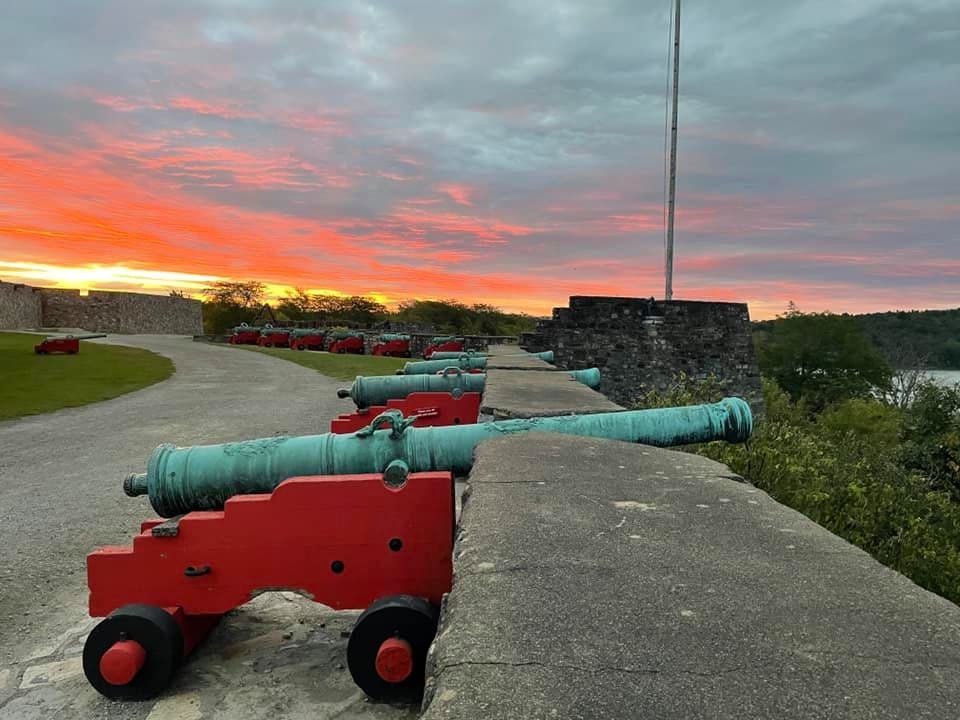The image captures an antique fortress at dusk, featuring several weathered cannons with a green patina seated in cement wells. These cannons, reminiscent of historical wars, are mounted on red and black wooden carriages equipped with wheels. A stone wall and a paved walkway curve along the left side of the scene, where one cannon is positioned solo. To the right, more cannons are aligned, pointing outward. Above this area stands a tall flagpole, though the flag is not visible. The sky is rich with reds and yellows from a picturesque sunset, with clouds adding depth and drama. In the background, beyond the cannons, a verdant trail meanders through green terrain, bordered by water and rolling hills. The setting vividly combines historical ambiance with the tranquil beauty of nature at day’s end.